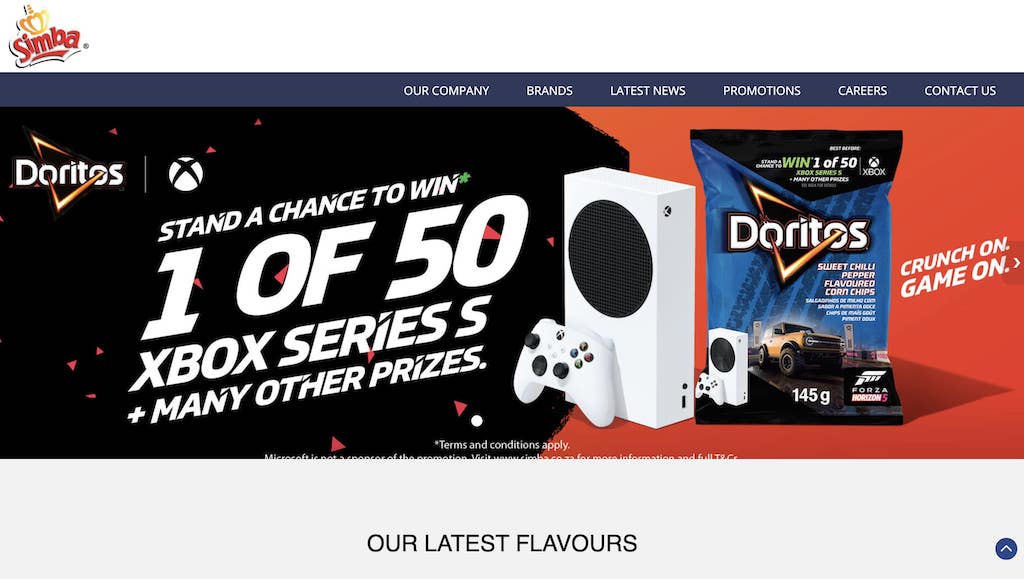Detailed Caption:

This is a promotional advertisement for Doritos, possibly from their website or an associated campaign page. In the upper left corner, there is a logo that reads "Simba," which appears in a yellow and red color scheme on a white background—a common branding seen in Asia. 

The page layout includes a horizontal navigation bar atop the main content, featuring dark blue bands with white text for categories such as "Our Company," "Brands," "Latest News," "Promotions," "Career," and "Contact."

The main image is a horizontally elongated graphic; the left half is predominantly black, transitioning to red on the right. In the upper left corner of this image, the Doritos logo is prominently displayed inside a triangular frame. Below the logo, a white circle with an 'X', which is indicative of Xbox, is paired with angled text stating, "Stand a Chance to Win 1 of 50 Xbox Series S plus many other prizes."

Visually, the promotion features an Xbox Series S console and game controllers, which are primarily white with black accents. Accompanying this are Doritos bags, specifically highlighting their "Sweet Chili Pepper Flavor Corn Chips." Both the product packaging and promotional text reiterate the chance to win the Xbox Series S and other prizes. The right side of the image boldly states, "Crunch On, Game On," connecting the snacking experience with an enhanced gaming session.